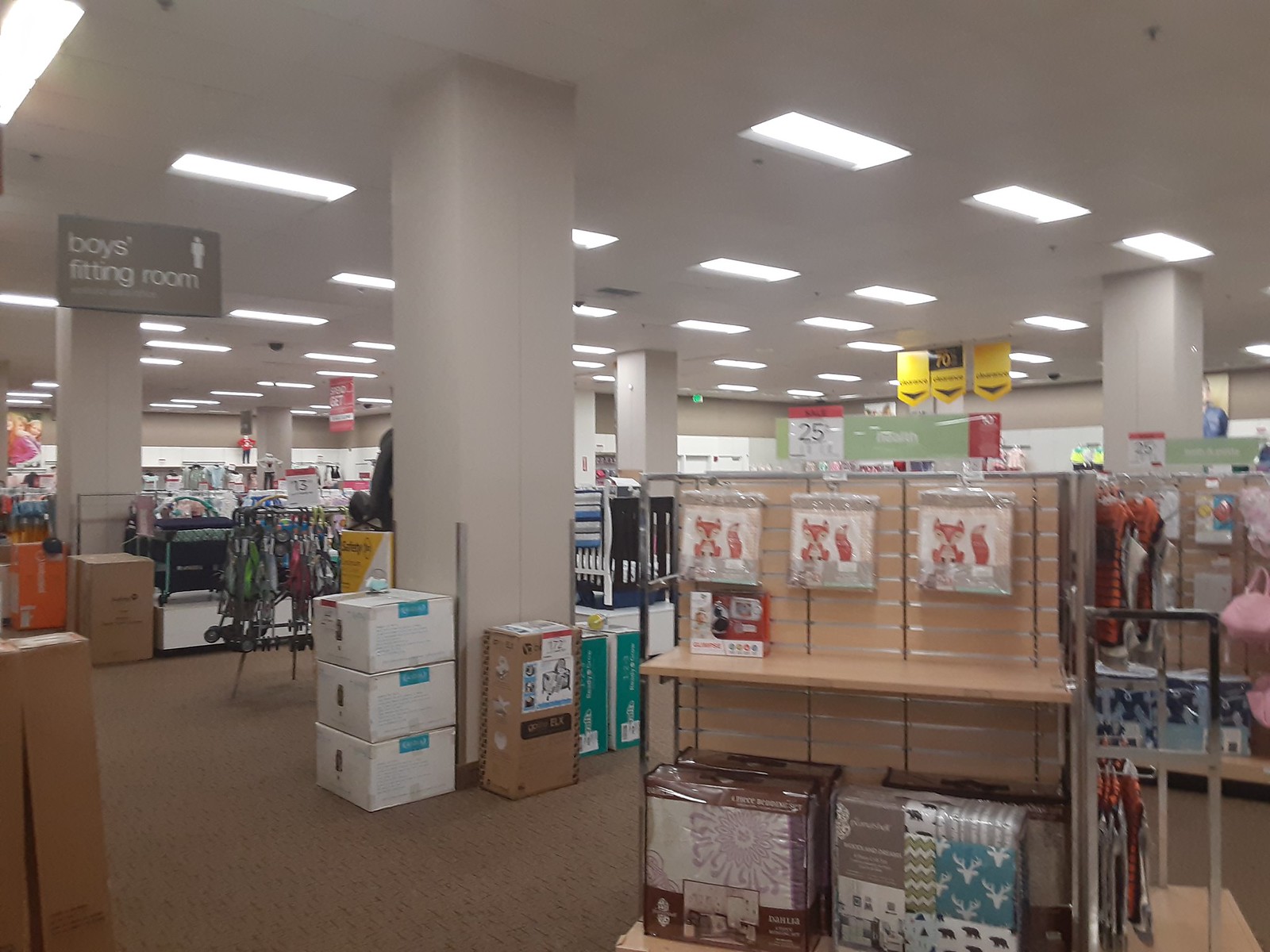The photograph captures the interior of a department store with a focus on both structural and display elements. The upper half of the image prominently features a ceiling of white tiles interspersed with rectangular fluorescent lights. Multiple white support beams, six in total, are spaced throughout the frame. In the upper left corner, a gray sign reading "Boy's Fitting Room" hangs from the ceiling, adorned with a white humanoid graphic in the upper right corner of the sign.

Beneath the ceiling, the store's layout becomes apparent. Beige carpeting covers the floor, leading up to a central display of comforters or bed sheets neatly arranged in plastic squares. Nearby, a support beam stands next to a stack of boxes. In the distance, towards the right side of the photograph, several yellow signs hang from the ceiling, although their text is not legible. The combination of these elements provides a comprehensive view of the store's organizational and structural details.